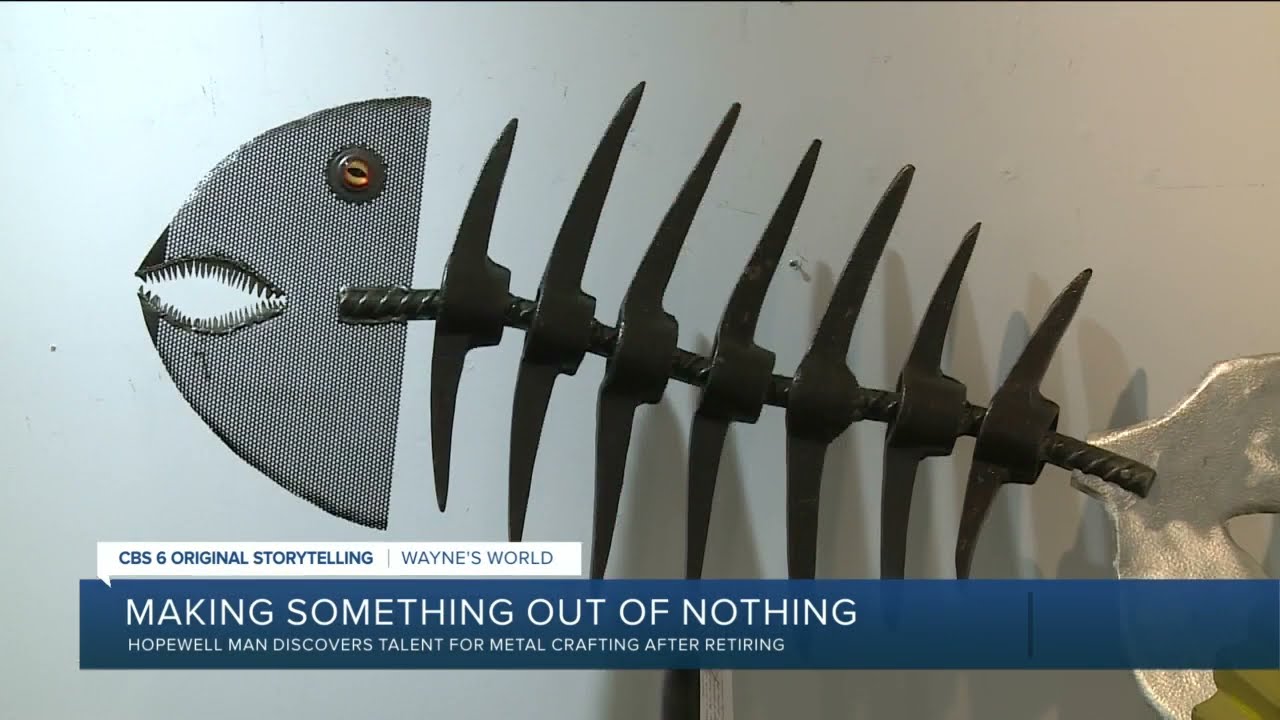In this detailed, landscape-oriented color photograph, a striking piece of metal artwork is showcased within the frame of a news broadcast. The image captures a dark gray metal sculpture of a fish skeleton against a light gray wall that transitions from a light aqua tone to a gentle tan hue. The fish's head is made from a mesh-like material, featuring a button for an eye and a zipper for teeth. Its body is constructed from metal strips resembling bones, culminating in a sculpted silver blob as the tail. At the bottom of the image, a dark blue rectangle with white text reads: "Making something out of nothing, Hopewell man discovers talent for metal crafting after retiring." Just above this, the chyron includes, "CBS-6 Original Storytelling/Wayne's World," with "Wayne's World" in blue text within a white conversation bubble pointing towards the main caption. This freeze-frame photograph from a local news broadcast vividly captures the intricate details of the unique sculpture, highlighting the artist's impressive craftsmanship.